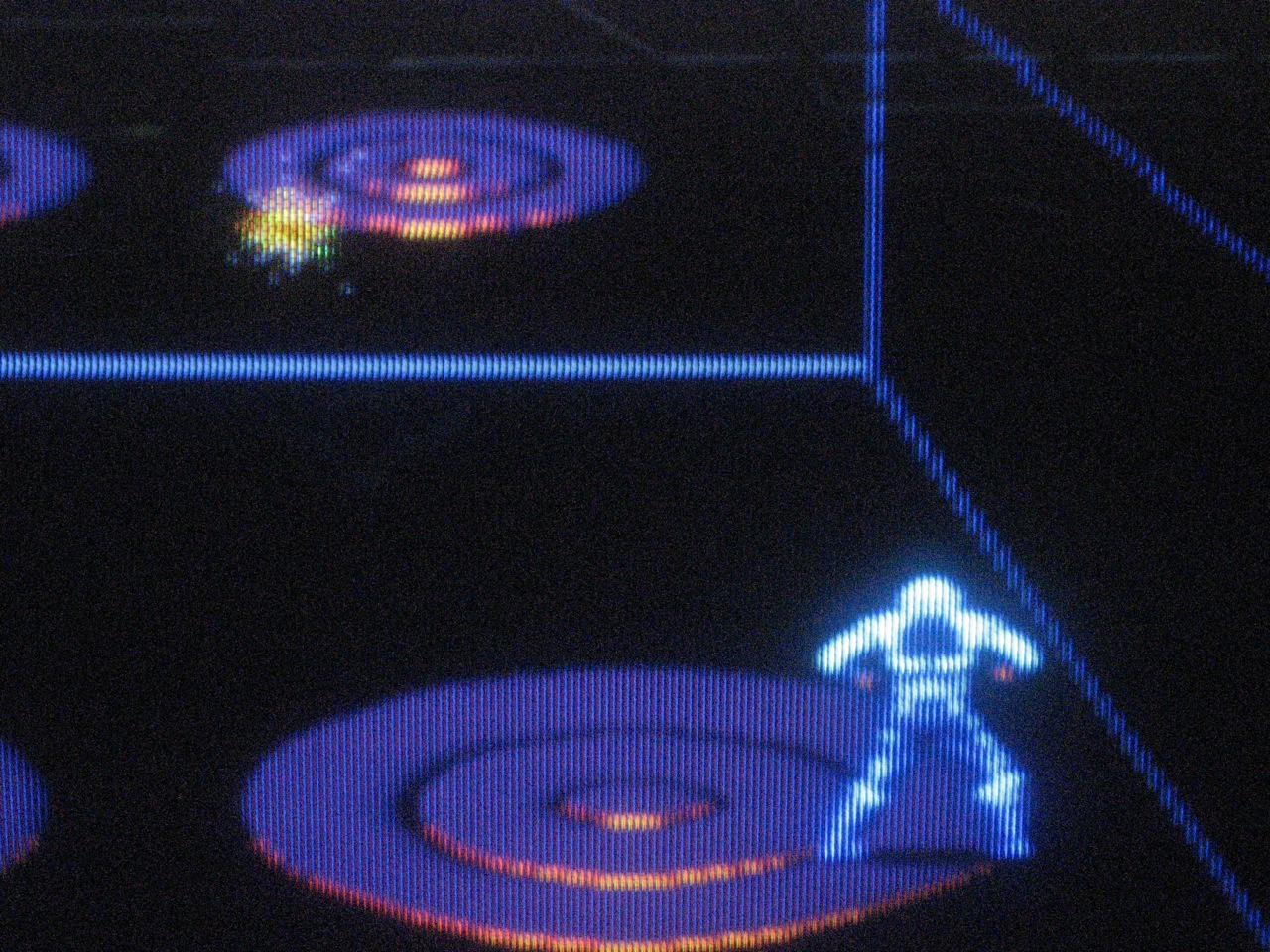The image is a detailed still from a pixelated video game, reminiscent of an old-school classic like Tron. At the bottom right corner, a central figure, likely the player character, stands in a dynamic combat pose on a glowing blue and white circle, which appears to be a high-tech transportation pad. The character is decked out in a bright blue and white suit of armor that emits a glowing aura, indicative of advanced technology or a space suit.

The room is defined by blue, glowing digital lines that outline the walls and create a Tron-like environment. There is another brighter circular pad visible in the background, suggesting a network of connected transportation points. Additionally, two faint circles can be seen on the far left side of the image.

In the background, near the glowing pad, a yellow and red pixelated shape suggests the presence of a potential adversary, possibly a monster or an alien entity. The overall scene is set against a dark, black backdrop, enhancing the vibrant neon colors and the pixelated retro aesthetic.